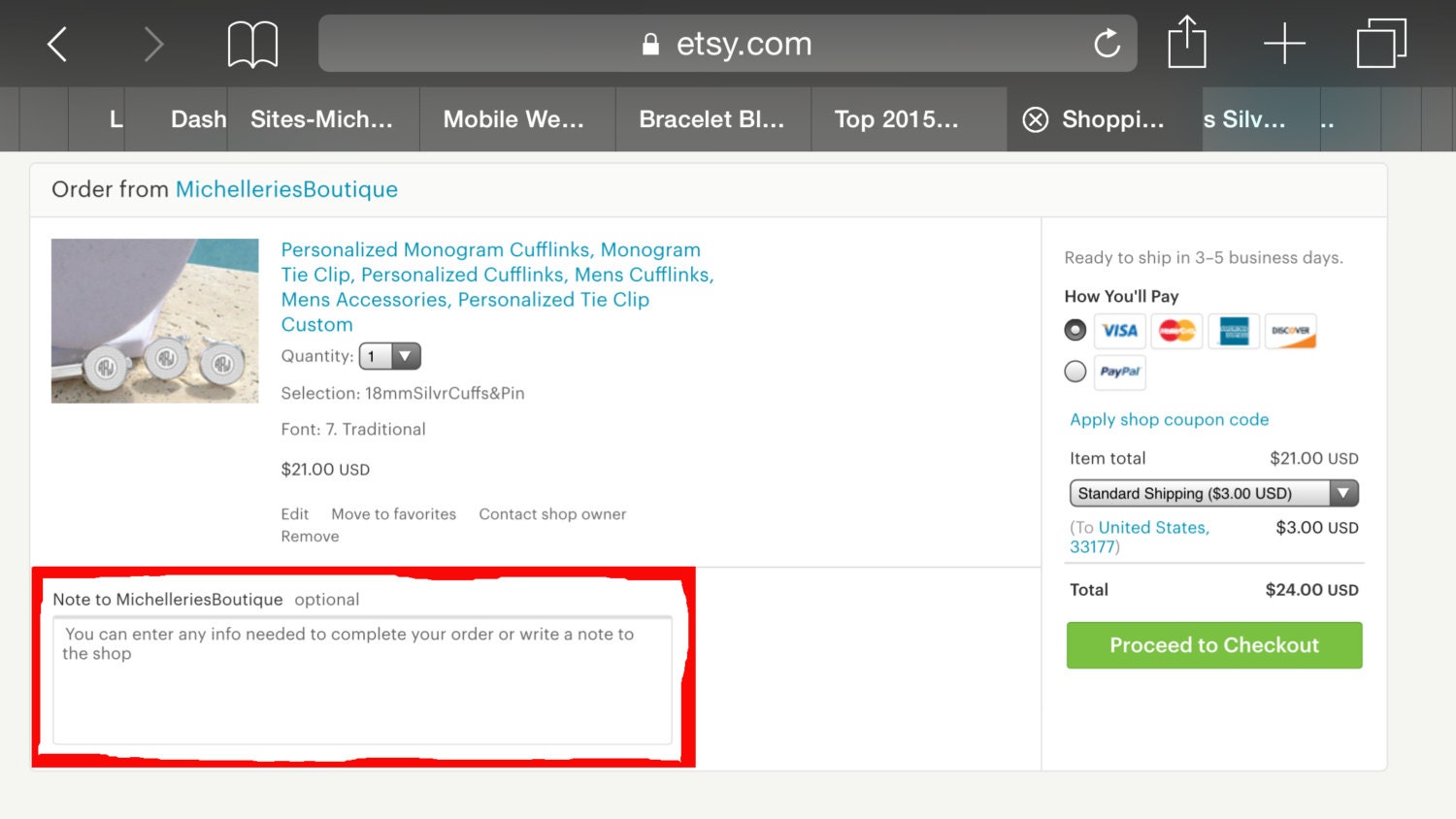**Caption:**

The image features a webpage, likely an Etsy shop. At the top, a white lock icon appears on a gray banner against a black background, signaling a secure site. Further down, there's a text entry starting with "L-sites-m-i-c-h…" and continues with "mobile w-e... bracelet bl... top 2015..." Next to it, a white 'X' and phrases like "shopping," "s-h-o-p-p-i..." and "s-l-s-i-l-v..." are seen.

Below that, the page transitions to a white section. On the left, it says "Order from" with "Michellerie's boutique" in blue. This is followed by product options listed in blue font: "Personalized monogram cufflinks," "monogram tie clip," "personalized cufflinks," "men's cufflinks," "men's accessories," "personalized tie clip," and "custom." Further down, in gray, the text reads: "Quantity," with an input field showing "1." The selection mentions "18 mm silver cufflinks" and "bin font seven traditional," priced at "$21 USD."

Options to "edit," "move to favorites," or "contact shop owner" are available. Additionally, there's a note field labeled "Note to Michellerie's boutique (optional)" highlighted in red with a box around it, instructing users to "enter any info needed to complete your order or write a note to the shop."

On the right, shipping information is provided: "Ready to ship in 3-5 business days." Payment methods listed include Visa, MasterCard, American Express, Discover, and PayPal, with each logo colored accurately. There’s also an option to "Apply shop coupon code."

At the bottom in black text, the "Item total" is "$21 USD" with a banner reading "Standard shipping (3 USD)." The shipping details show "To United States 33177 (3 USD)." The grand total is "$24 USD." Finally, a green banner at the very bottom reads "Proceed to checkout" in white.